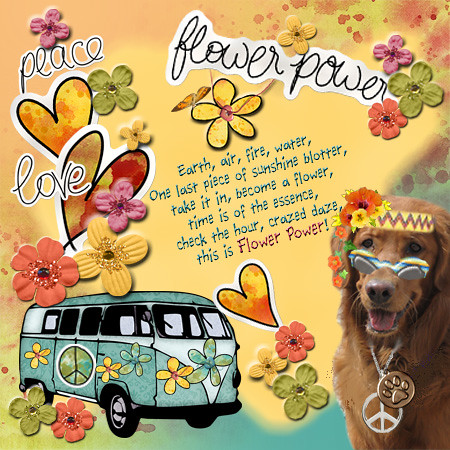The image is a vibrant, detailed flyer themed around "Flower Power," peace, and love. Dominated by bright yellows and blues, it features a colorful array of hearts and various flowers sprinkled throughout. The central message reads: "Earth, air, fire, water, one last piece of sunshine, blotter. Take it in, become a flower. Time is of the essence, check the hour. Craze days, this is flower power."

A prominent element in the image is a greenish Volkswagen bus adorned with yellow and green flowers, peace symbols, and multiple windows. In the bottom right corner, a dark brown collie dog is superimposed, wearing sunglasses and decorated with both a dog necklace and a peace sign necklace, surrounded by more flower embellishments. The flyer is divided into a yellow upper section and a light blue lower section, featuring yellow and red hearts, as well as flowers in shades of green, pink, and orange. Overall, the image conveys a nostalgic, hippie-era vibe celebrating peace, love, and nature.